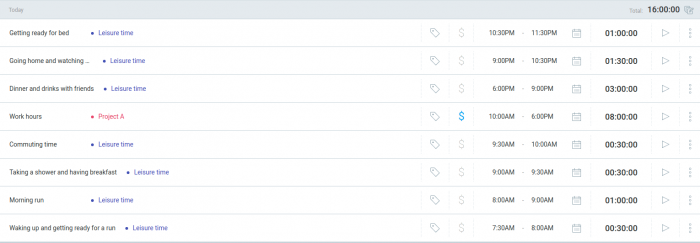This image depicts a website with a structured daily schedule, though the text is challenging to read due to its small size. The top part of the website features a gray bar with "Today" on the left side, and on the right side, it reads "Total: 16:00:00," accompanied by a copy icon. Below this bar, the schedule is divided into eight vertical sections, each representing specific activities. The activities and their corresponding colors are as follows:

1. Get ready for bed - Leisure time (purple)
2. Going home and watching... - Leisure time (purple)
3. Dinner and drinks with friends - Leisure time (purple)
4. Work hours, Project A (red)
5. Commuting time - Leisure time (purple)
6. Taking a shower and having breakfast - Leisure time (purple)
7. Morning run - Leisure time (purple)
8. Waking up and getting ready for a run - Leisure time (purple)

To the right of this main section, there are additional columns, each containing specific icons and details:

- The second column contains bookmark icons next to each activity.
- The third column displays dollar signs for each activity, with the dollar sign for the work hours section highlighted in blue.
- The fourth column lists the times for each activity in the following order: 
  - 10:30 p.m. to 11:30 p.m.
  - 9 p.m. to 10:30 p.m.
  - 6 p.m. to 9 p.m.
  - 10 a.m. to 6 p.m.
  - 9:30 a.m. to 10 a.m.
  - 9 a.m. to 9:30 a.m.
  - 7:30 a.m. to 8 a.m.
- The fifth column shows the duration of each activity:
  - 1 hour
  - 1 hour 30 minutes
  - 3 hours
  - 8 hours
  - 30 minutes
  - 30 minutes
  - 1 hour
  - 30 minutes
  - The next column has a play button icon next to each time slot.
- The sixth column has a calendar icon for each activity.
- The final column is represented by three dots next to each item.

The layout is intended to provide a detailed, organized view of a day's schedule, categorizing all activities using color-coded leisure time and work segments.